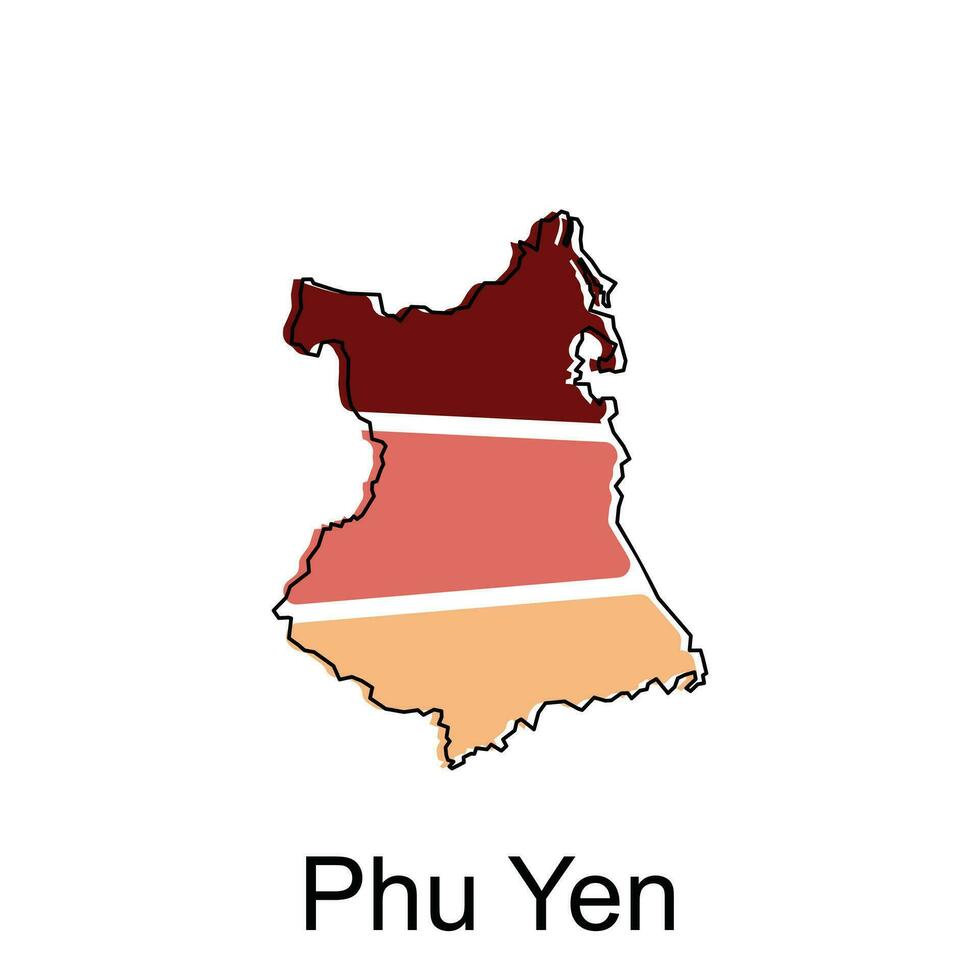The image depicts a detailed and creatively illustrated map of Phu Yen, a province in Vietnam. The map is divided into three horizontal sections, each distinctly color-coded. The top section is a deep burgundy, the middle section is salmon or deep peach, and the bottom section is a light beige. These segments are separated by thin white lines. The entire map, which is tall and slender, is outlined in black ink, emphasizing its irregular shape. Above this colorful depiction, the name "Phu Yen" is spelled out in large black letters, with "P-H-U" and "Y-E-N" separated by a space. A minimalistic silhouette of Vietnam is present above the text, reinforcing the geographical context. This artistic representation likely uses color to distinguish different areas within the region.